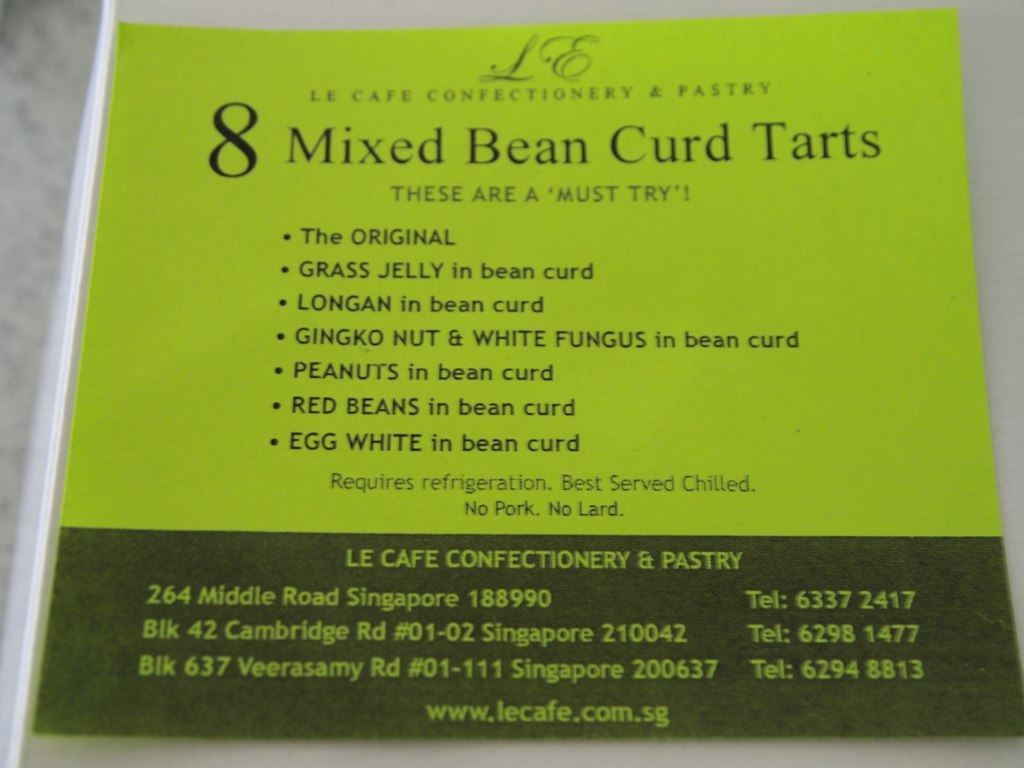A promotional flyer printed on bright lime green paper for Le Café Confectionary and Pastry. At the top, in elegant cursive, are the letters "L" and "E". Beneath, in a large black serif font, the text reads "Le Café Confectionary and Pastry". Below that, in even larger black text, it states "8 Mixed Bean Curd Tarts" with a smaller caption underneath that declares, "These are a must-try!" Following this, there is a detailed bulleted list of tart varieties:
1. Original
2. Grass Jelly and Bean Curd
3. Longan and Bean Curd
4. Ginkgo Nut, White Fungus, and Bean Curd
5. Peanuts and Bean Curd
6. Red Beans and Bean Curd
7. Egg White and Bean Curd

Additional notes beneath the list in lighter black text mention:
- Required Refrigeration
- Best Served Chilled
- No Pork

At the bottom of the flyer, a black background section with green text reiterates the café's name and provides three Singapore addresses with corresponding details:
1. 264 Middle Road, Singapore, 188990
2. BLK 42 Cambridge Road, #01-02 Singapore, 210042
3. BLK 637 Veerasamy Road, #01-111 Singapore, 200637

The website is listed as www.lecafé.com.sg. On the bottom right corner, several contact numbers are provided: TEL 63372417, TEL 62981477, and TEL 62948813.